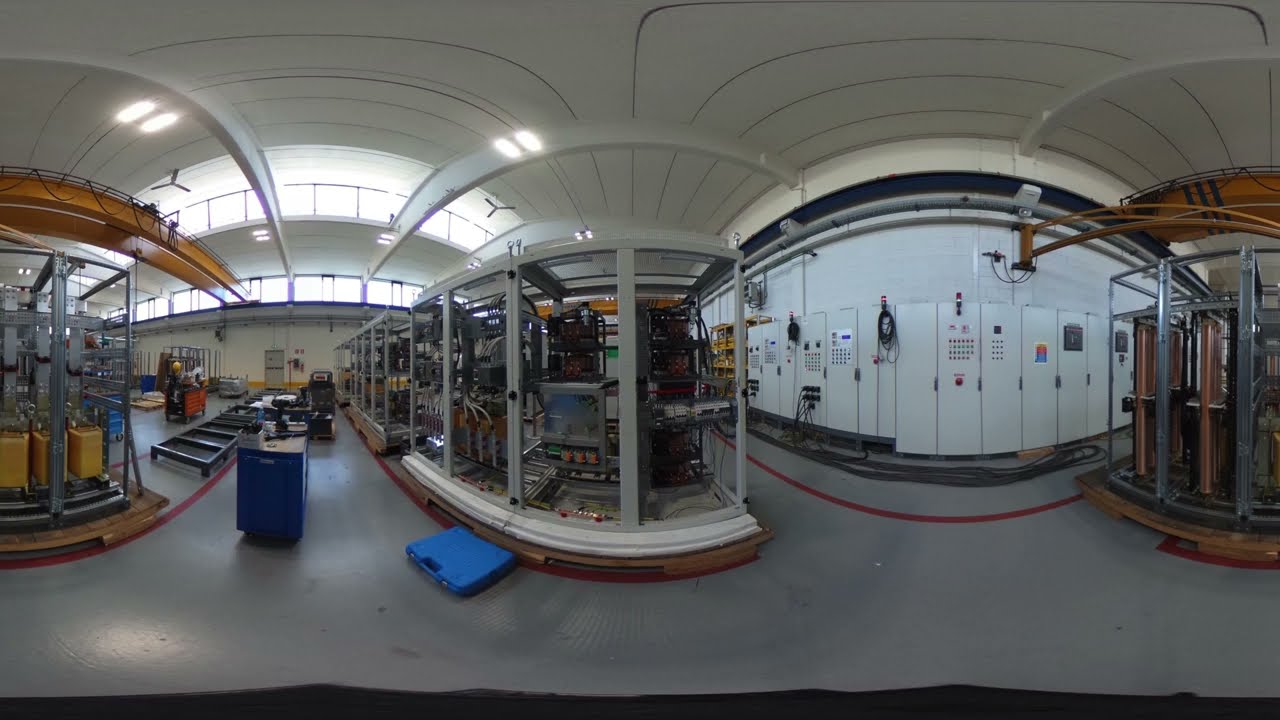The image depicts the interior of a modern factory or machine shop characterized by enclosed areas with glass paneling, allowing a clear view of the computers and machinery housed within. The concrete floor features a blue toolbox positioned in the central section, directly in front of one of these enclosed areas. To the left, amidst various equipment, a ladder lies on the floor next to some electrical plugs and wires protruding from the wall. Above this, an upper level with glass windows overlooks the workspace below. The factory's white walls and ceiling are supported by distinctive curvy beams, and windows in the background allow natural light to filter in. On the right, white electrical panels are visible, indicative of the workspace's technical and operational focus. The environment suggests a high-tech facility dedicated to manufacturing or electronic maintenance, with shelves and workbenches supporting the intricate machinery and electronic equipment.